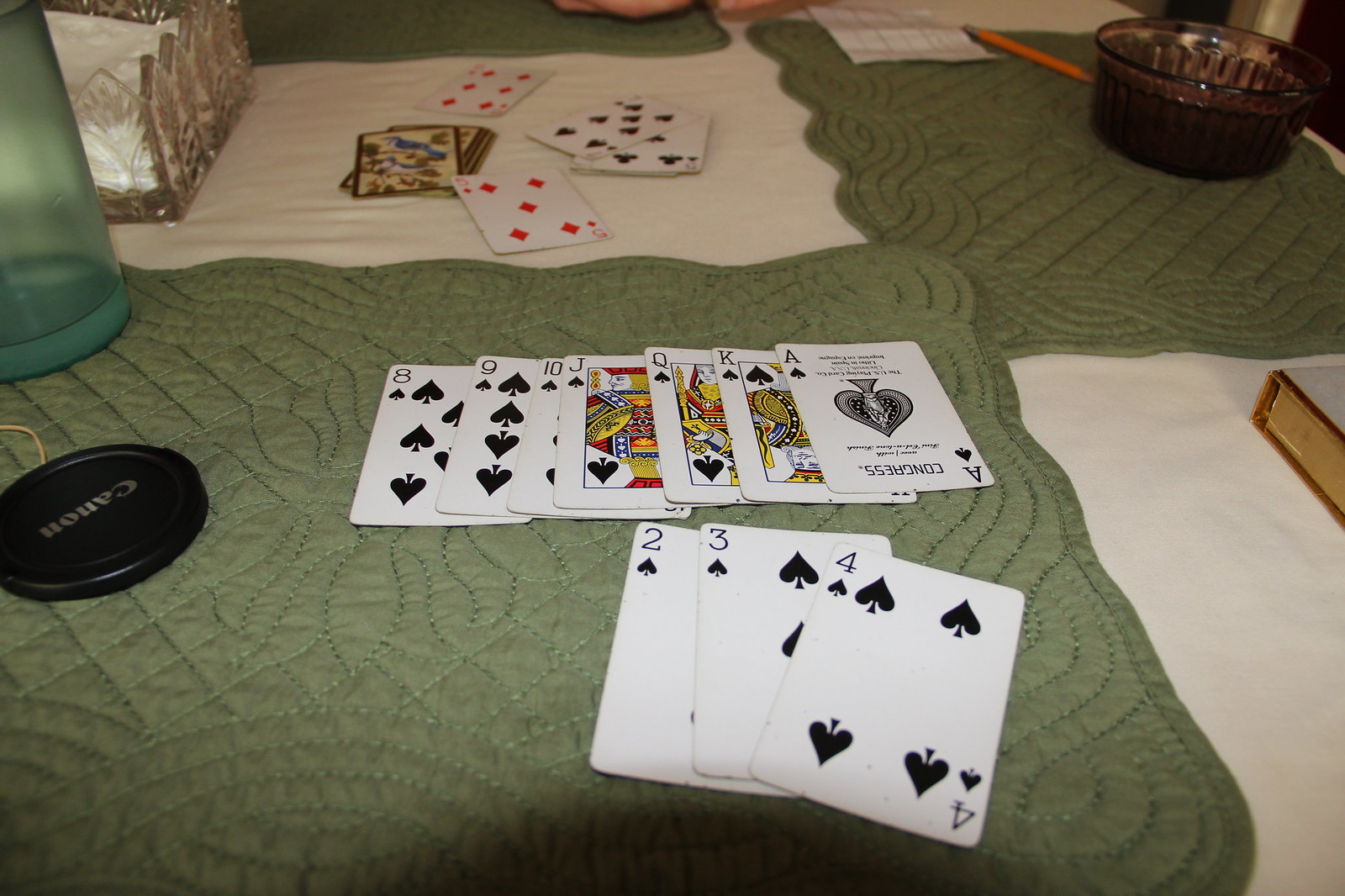On a pea green coffee table with dark green stitching lies a clear arrangement of playing cards. In the center, the 8, 9, 10, Jack, Queen, King, and Ace of Spades are prominently displayed in sequence. Below this sequence, the 2, 3, and 4 of Spades are spread out in a neat row. To the right, there is a white cloth partially covering a book with brown trim, gold-edged pages, and a white cover. Behind this book, a brown crystal glass is positioned next to what appears to be an ashtray holding a yellow pencil. Further along, some scattered papers add to the scene's casual clutter.

Next to another white cloth, the 5 of Diamonds and several cards featuring both Spades and Diamonds are laid out. Intermingled among these face-up cards is a small stack of face-down cards, roughly half or a quarter of a deck. Towards the left, a gold metal shelf holds an assortment of white papers. Adjacent to this shelf sits a clear bottle and a black plastic object labeled "Canon" in light gold lettering, with a piece of a rubber band lying beside it. The scene suggests an engaging, yet casual card game in progress, accompanied by an array of personal items.